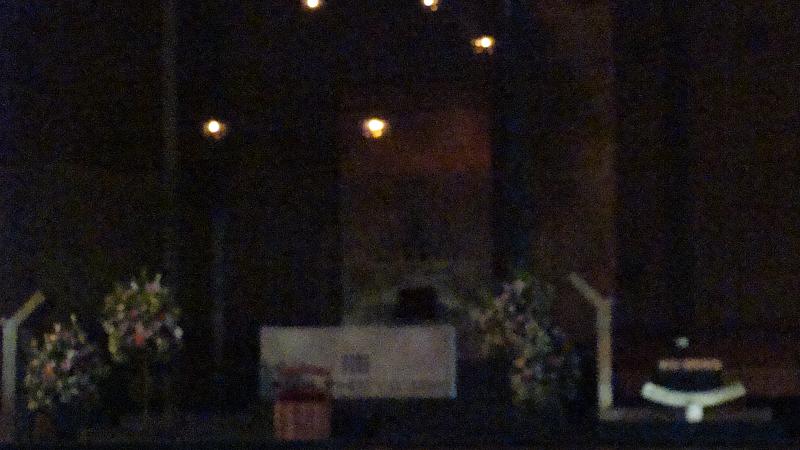The image, captured outdoors at night, is grainy and dark. In the upper portion of the photograph, numerous lights are visible, seemingly attached to the exterior of a stone or brick building. The building's facade is partially landscaped, featuring what appears to be a tree or bush near the entrance. In front of the building, there is a rectangular sign mounted on a striped platform, though the blue print on the sign is illegible. Additionally, two small, manicured trees are positioned to the left side of the image.